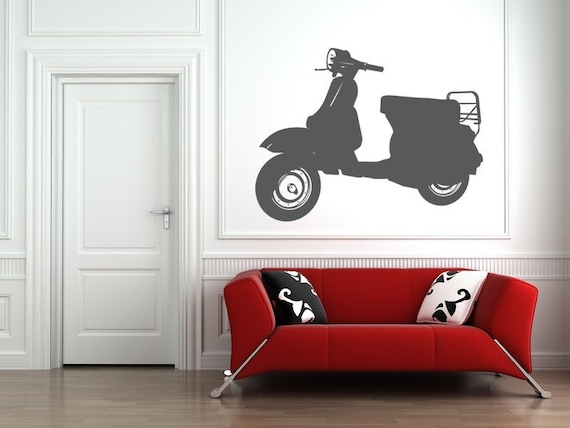The image depicts a brightly lit hallway-like room with a pale brown wooden floor featuring horizontally aligned panels. Dominating the right side of the image is a small red couch with integrated cushions that appear fixed to the structure. The couch, suitable for one or two people, has angled metallic legs extending outward from the middle of the seat. Adorning the couch are two matching pillows with opposite designs: a black pillow with white patterns on the left, and a white pillow with black patterns on the right. Above the couch hangs a framed monochromatic artwork depicting a black and white moped with some gray shading, creating a silhouette-like effect against the white background. To the left of the couch is a closed white door equipped with a stainless steel handle, complementing the room's white walls and adding to the bright and clean ambiance. No people are visible in the image.